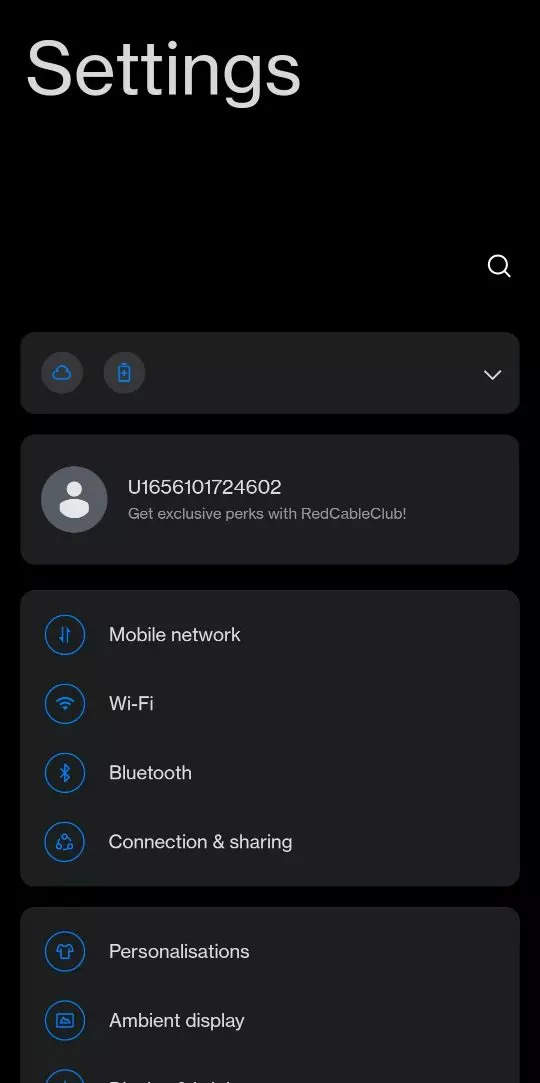This image, captured from a smartphone's settings page, predominantly features a black background. At the top, the word "Settings" is displayed in white, with the 'S' capitalized and the remaining letters in lowercase. On the right side of the screen, there is a magnifying glass icon indicating a search function.

Scrolling down, two icons are visible: one representing a cloud and another showing a battery. Further down, a clickable drop-down menu is presented within a rectangle.

The next section of the screen includes a white silhouette of a human figure placed inside a gray circular background. Accompanied by a long alphanumeric code, it contains the text "Get exclusive perks with Red Club."

Continuing down, there is another rectangle housing four icons, each tipped with blue but primarily black. These icons are labeled as follows: "Mobile Network," "Wi-Fi," "Bluetooth," and "Connection and Sharing."